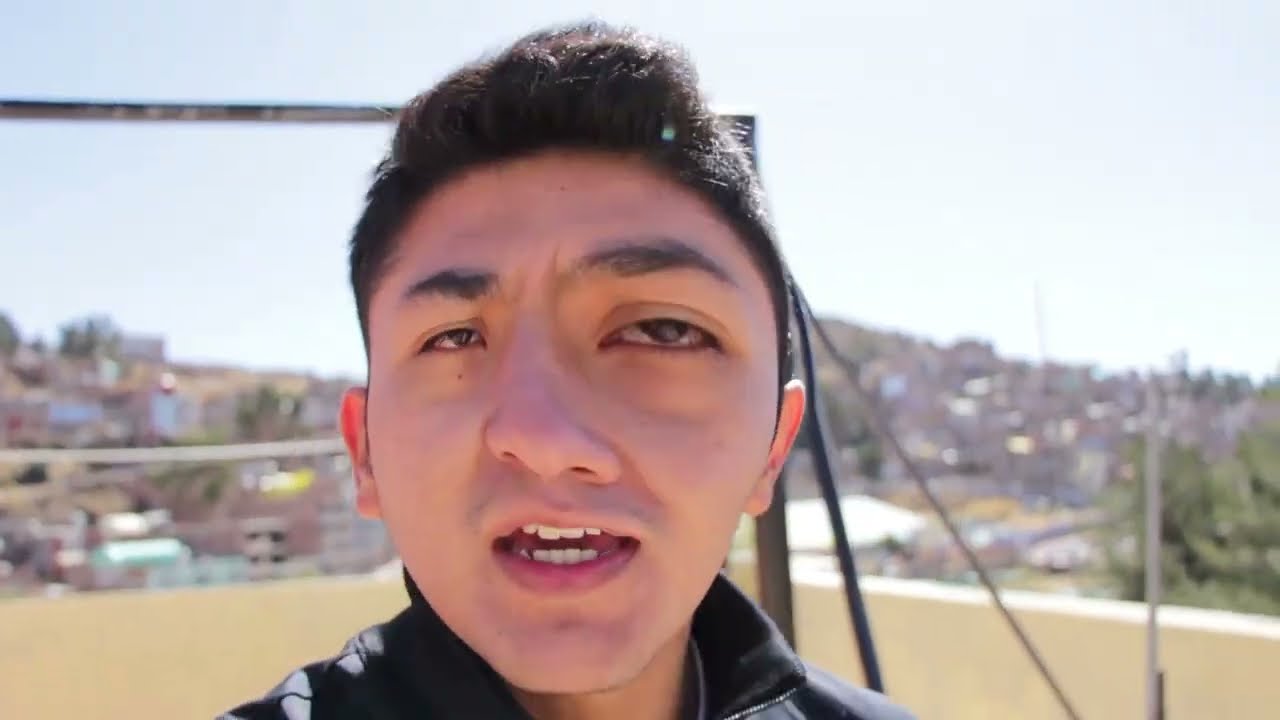The image depicts a close-up headshot of a man who appears to be of Hispanic or Latin American descent, characterized by his short black hair and light to brown skin tone. He is clad in a black sweater, and his background showcases a densely built, multicolored, favela-style city set against a clear blue sky. The man seems to be standing at an elevation, possibly on top of a building, overlooking a sandy field that precedes the blurred cityscape. The photo features a noticeable distortion, as the left side of his face appears normal while the right side is heavily warped and blurred, likely due to a Photoshop effect. This effect causes his right eye to be abnormally large, his nose to bend unnaturally, and his cheek and chin to bow outward, giving his face an overall disfigured appearance.